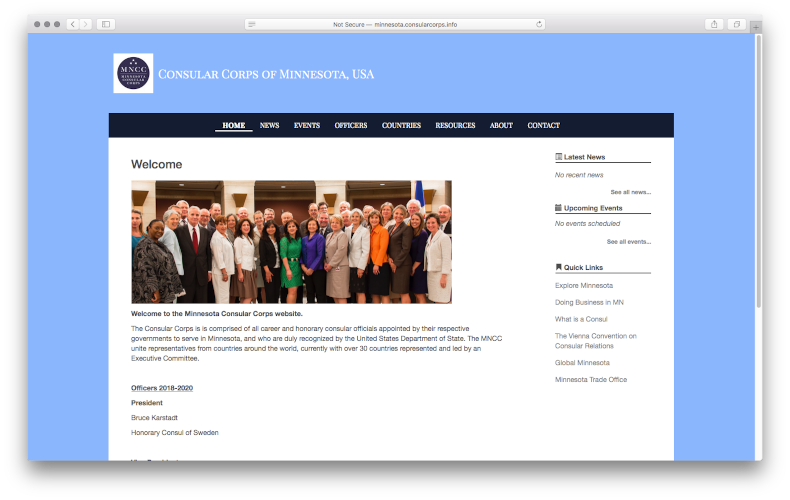The image showcases the homepage of the Consular Corps of Minnesota, USA's website. 

At the top, a gray border spans the width of the page. On the top left of this border, there are three dots followed by left and right arrow icons, along with another small, indiscernible symbol. Centrally located within this border is what appears to be a search bar, labeled "Not Secure" and displaying the URL, "Minnesota, ConsulCorps.info." On the top right, there are additional icons that seem to facilitate actions like downloading or enabling picture-in-picture mode.

The main background of the page is light blue. Centrally positioned and stretching towards the bottom, there is a section bordered in black at the top with a white background within. Above this section, in white text, it reads "Consular Corps of Minnesota, USA." Adjacent to this, on the left, there is a small white square containing a blue circle with some minute, unreadable letters inside.

Below this header, a black navigation banner features links labeled "Home," "News," "Events," "Officers," "Countries," "Resources," "About," and "Contact."

In the section with the white background, the word “Welcome” appears in the upper left corner. Below this, an image shows a group of men and women standing together. Underneath the picture, there is a brief synopsis, containing several small, hard-to-read words, including the President's name. On the right side of this section are headings such as "Latest News," "Upcoming Events," and "Quick Links," providing additional navigational options and information.